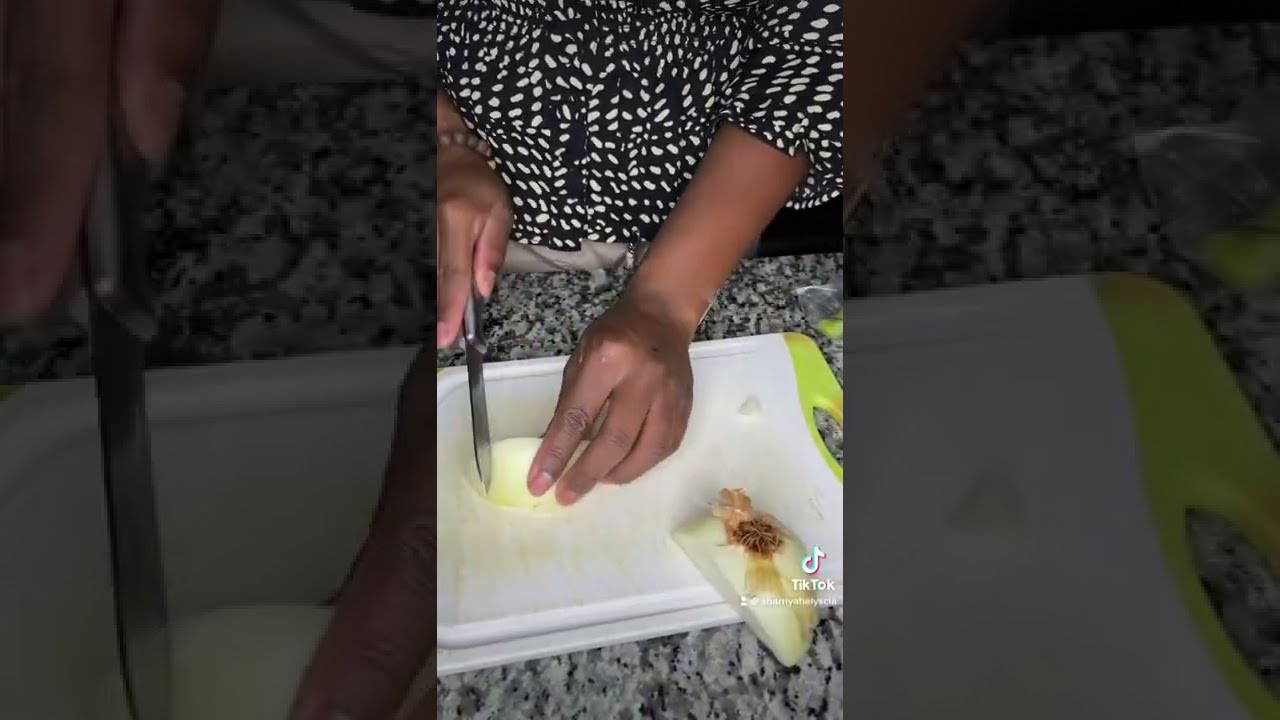This is a vertical photograph from a cell phone, capturing a screenshot of a TikTok video. The central image is a close-up of a dark-skinned woman’s hands and partial torso as she cuts an onion. She is wearing a black blouse adorned with white polka dots. Her left hand holds a section of the onion, ready for slicing, while her right hand steadies a knife. The onion rests on a white plastic cutting board with a bright green handle, positioned on a black and white marble countertop. A partially sliced onion, with the stem still attached, is also visible beside the cutting board on the lower right-hand side, near the TikTok logo. The overall scene is framed by darkened and enlarged portions of the image's central focus. The woman's left wrist features a beaded bracelet, and she is possibly wearing khaki pants, though only a part of her chest and abdomen are visible in the frame.